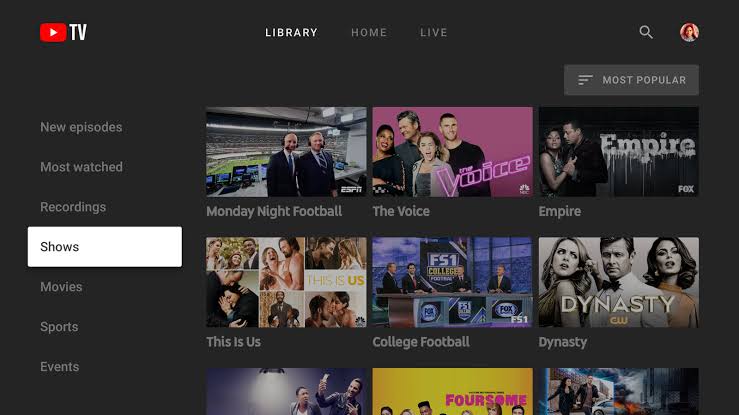The image is a screenshot from the YouTube TV app. At the top left corner, it prominently features the YouTube play button icon followed by the word "TV" in white font. Central to the top menu bar are three distinct tabs labeled "Library," "Home," and "Live," with the "Library" tab highlighted in white, indicating it is currently selected. 

On the left-hand side of the interface, there is a vertical navigation menu listing various categories: "New Episodes," "Most Watched," "Recordings," "Shows," "Movies," "Sports," and "Events." 

The main content area displays a series of selections under the categories within the Library tab. Notable highlighted shows and events include "Dynasty," "College Football," "The Voice," and "Empire." 

Each of these elements is laid out in a clean, user-friendly interface, characteristic of the YouTube TV app, making browsing through different categories and selections intuitive and visually appealing.